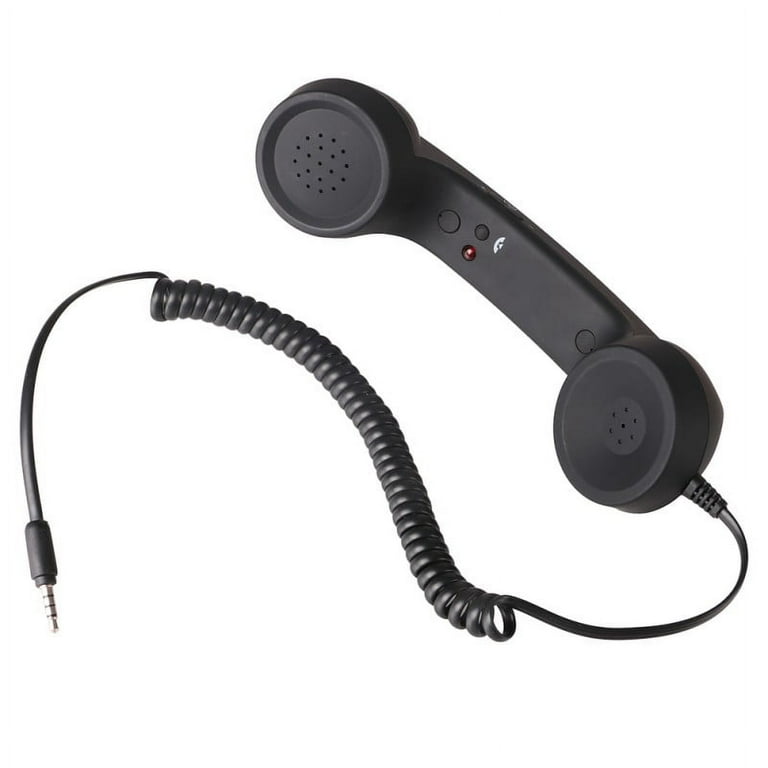The image showcases a vintage-style, black landline telephone receiver prominently placed at the center against a plain white background. The receiver, characterized by its minimalistic design, includes a single button marked with a symbol of a handset and a red LED light. A black spiral cord is attached to the receiver, resembling a coiled slinky, leading to an audio jack with a chrome pin at its end. The product lacks any labeling text, emphasizing its stark, old-fashioned aesthetic, which harks back to a bygone era of technology.